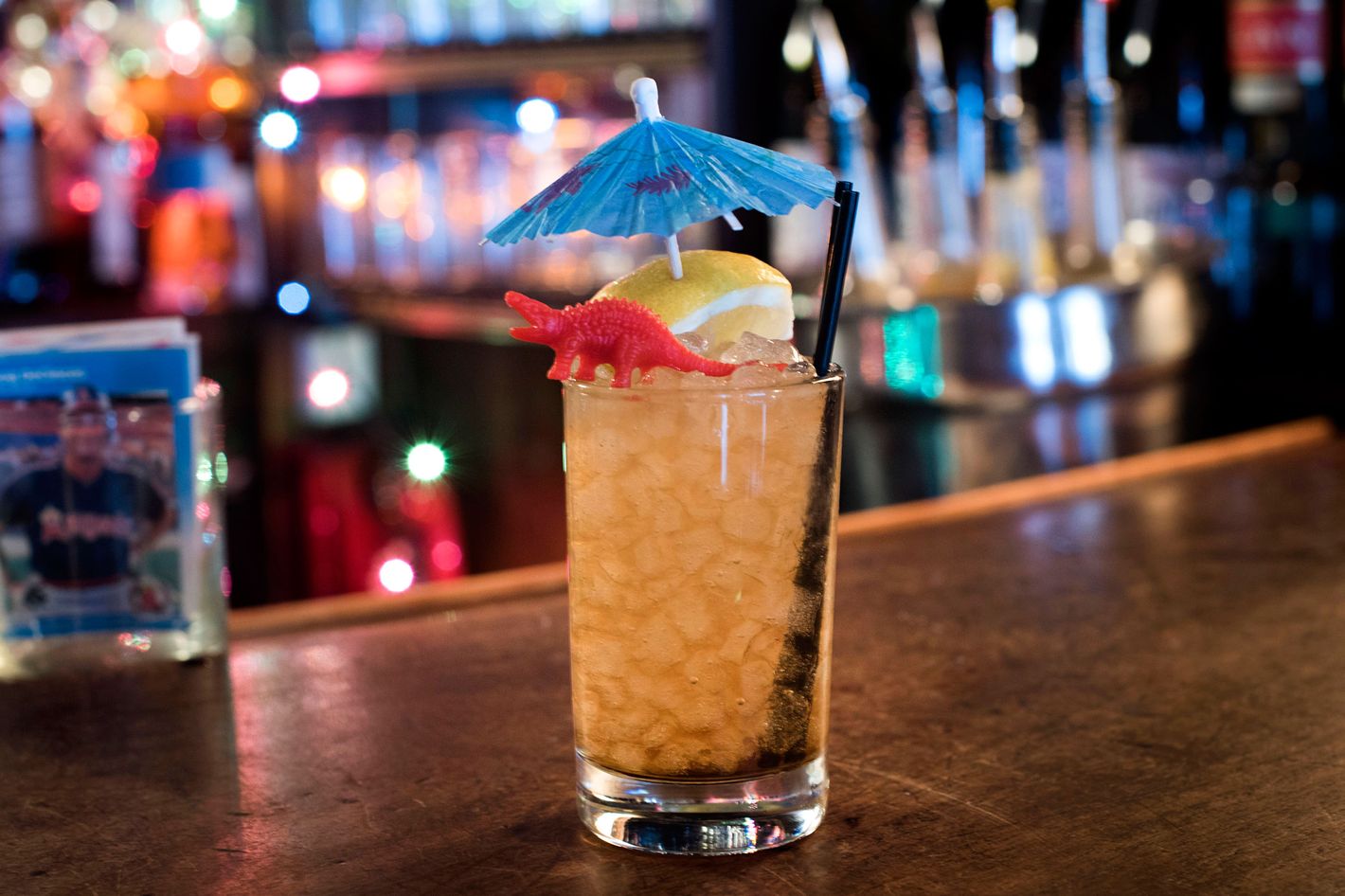In this vibrant landscape-oriented photograph taken inside a bar, the focal point is a tall, transparent glass of cocktail resting on a brown wooden bar. The cocktail, a light golden peach color, is filled to the brim with tiny ice cubes. Protruding from the glass are two thin black straws on the right and a lemon wedge garnished with a distinctive blue umbrella with purple leaves, making for a whimsical decoration. Adding a playful touch, a small red alligator or dinosaur figure clings to the top left rim of the glass. In the blurred background, the bar comes to life with bright lights gleaming in shades of blue, pink, and red, illuminating rows of liquor bottles and creating a festive atmosphere reminiscent of Christmas lights. To the left of the glass, a baseball card in a holder is set on the bar, while the upper right-hand corner features a blurred cake with a red label.